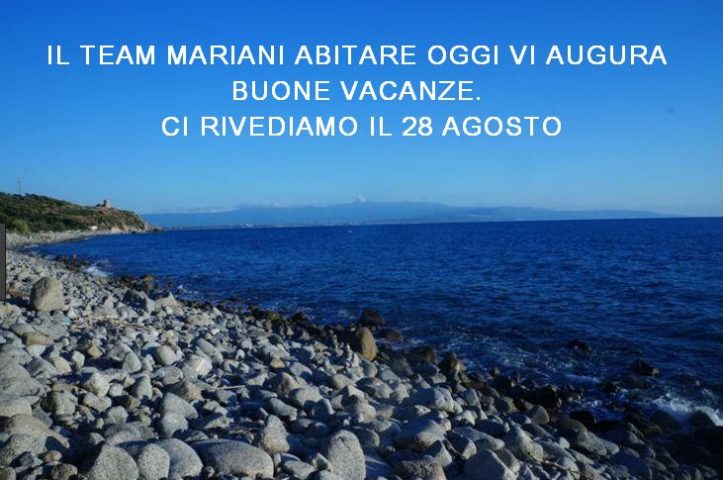The image depicts a serene rocky shoreline with light gray rocks scattered along the beach. The water transitions from a light blue near the shore to a darker blue further out. Small waves gently lap against the rocks. The backdrop features hazy mountains, likely due to heat haze, in the center and far distance. Midway on the left side, a green foliage-covered inlet is visible. The sky above is blue, and along the top of the image, there is text in what appears to be Italian, with phrases like "IL-10," "Mariani," "Arbitar," "Ogai V. Argar," "Buena Vaccine," "Remy Valdo," "IL-28," and "Augusto." The overall setting is outdoors, capturing the natural beauty of this coastal scene.